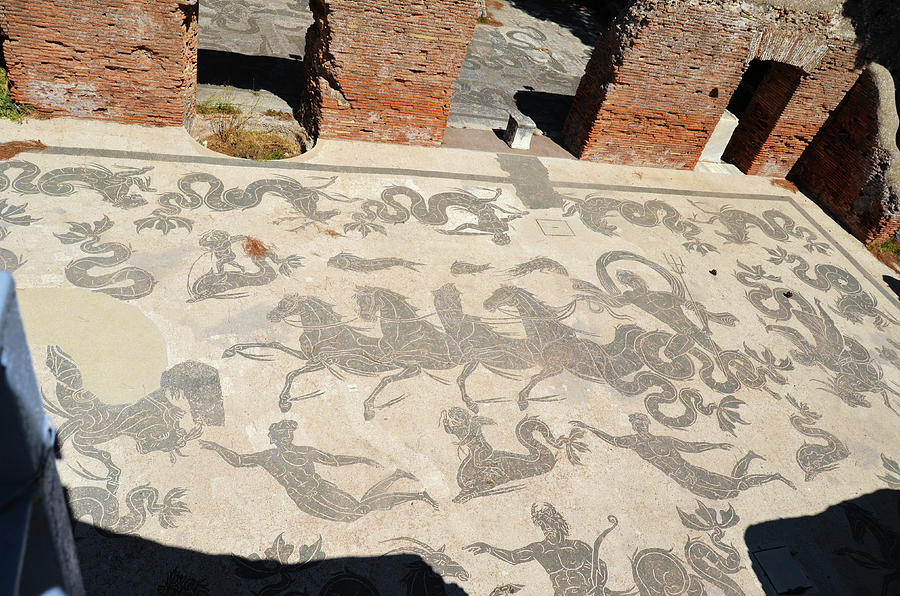The photograph captures an overhead view of an ancient archaeological site featuring a beautifully decorated floor with a light stone background, ranging in colors from light brown to creamy beige. The floor is intricately engraved with dark gray depictions of various creatures and people. Central to the composition is a line of four chariot horses, driven by a man on the right holding what appears to be a pitchfork or trident. Surrounding the horses are numerous detailed figures: serpents or snakes occupy the top and sides, while below the horses, there's a depiction of what appears to be a mermaid. Additional human figures can be seen swimming beneath the horses, including one riding a dolphin. The scene is framed by red brick columns and crumbling brick walls that highlight the ancient and ruinous nature of the site. An archway is visible to the right, enhancing the historical ambiance. Two shadows cast across the bottom corners of the image add a subtle touch of depth.